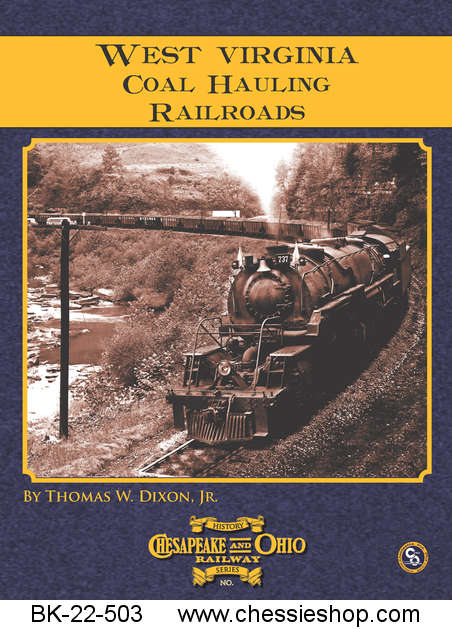The front cover of the book, titled "West Virginia Coal Hauling Railroads," features a prominently detailed yellow banner at the top with blue text. Beneath the banner, a black-and-white photo, tinted with sepia tones, captures a historic steam engine pulling multiple carts in a C-shaped curve through a mountainous landscape. The deep, dark grayish-purple background of the cover contrasts with the goldish-yellow border surrounding the evocative image of the train. This image imparts an aged charm, emphasizing the historical significance of coal transport in the region. The cover also includes blue text detailing "Chesapeake and Ohio Railway Series Number" and provides purchasing information at the bottom with the code "BK-22-503" from www.chessyshop.com. Authored by Thomas W. Dixon, Jr., this publication is a part of a dedicated series exploring the rich history of railroads.